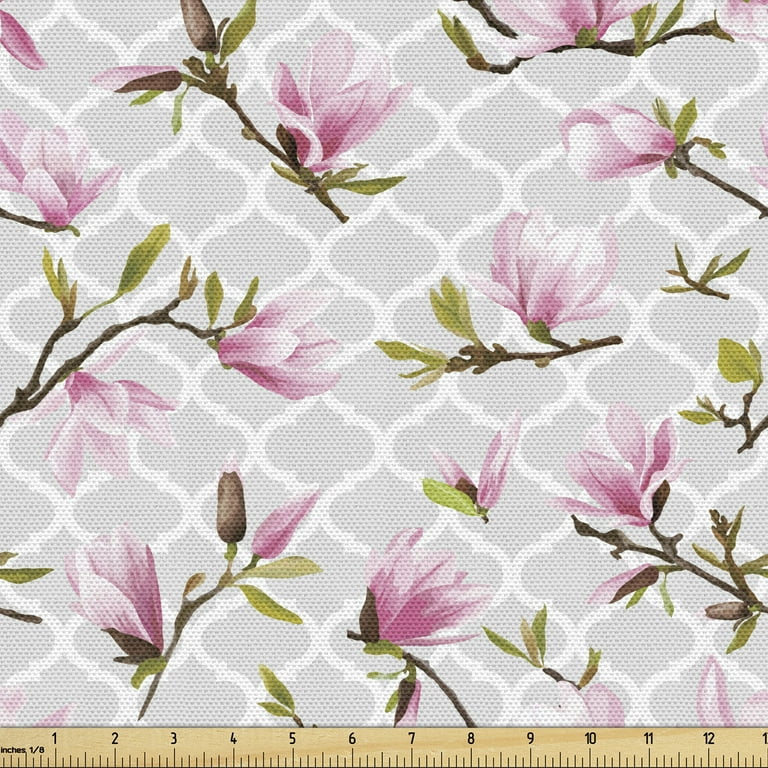Displayed in the image is a 13-inch wide square swatch of material that bears a striking resemblance to wallpaper or possibly canvas. The material has a light gray to orchid background adorned with a white pattern that appears to form diamond or four-leaf clover shapes. Overlaid on this patterned background are brown stems with green leaves and a variety of pinkish-purple flowers, depicted in different stages of growth. The flowers and stems contribute to a collage-like effect, accentuated by small darker dots scattered across the fabric. At the bottom of the image, a wooden ruler is positioned horizontally, marked with clear measurements from 0 to nearly 13 inches, confirming the size of the material. The intricate combination of patterns and natural elements creates a visually appealing and detailed composition.